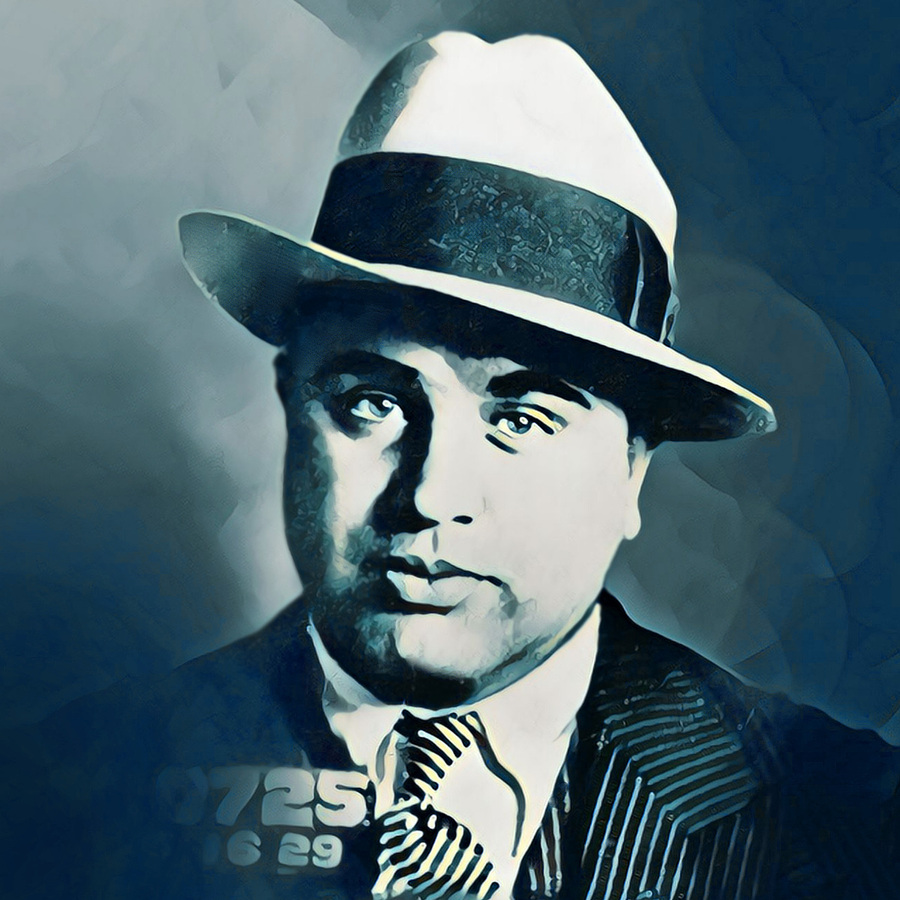This is a highly detailed and partially colorized portrait of the infamous gangster Al Capone, likely derived from a historic mugshot. The image primarily appears in black and white tones but features subtle hues of blue and streaks of yellow, particularly on his striped tie. Capone is depicted wearing a white fedora with a black band, a white shirt, and a heavily pinstriped suit typical of the 1920s. He is looking directly into the camera with a neutral expression, neither smiling nor frowning. The portrait, rendered in a Photoshop graphic design style, shows Capone from the chest up, with the background transitioning from lighter gray on the left to darker gray on the right. Over his right chest area, there are arrest numbers partially visible: 072 and smaller digits below reading 1629. The overall piece gives the impression of a blurred, liquefied effect, enhancing its vintage and somewhat eerie feel.